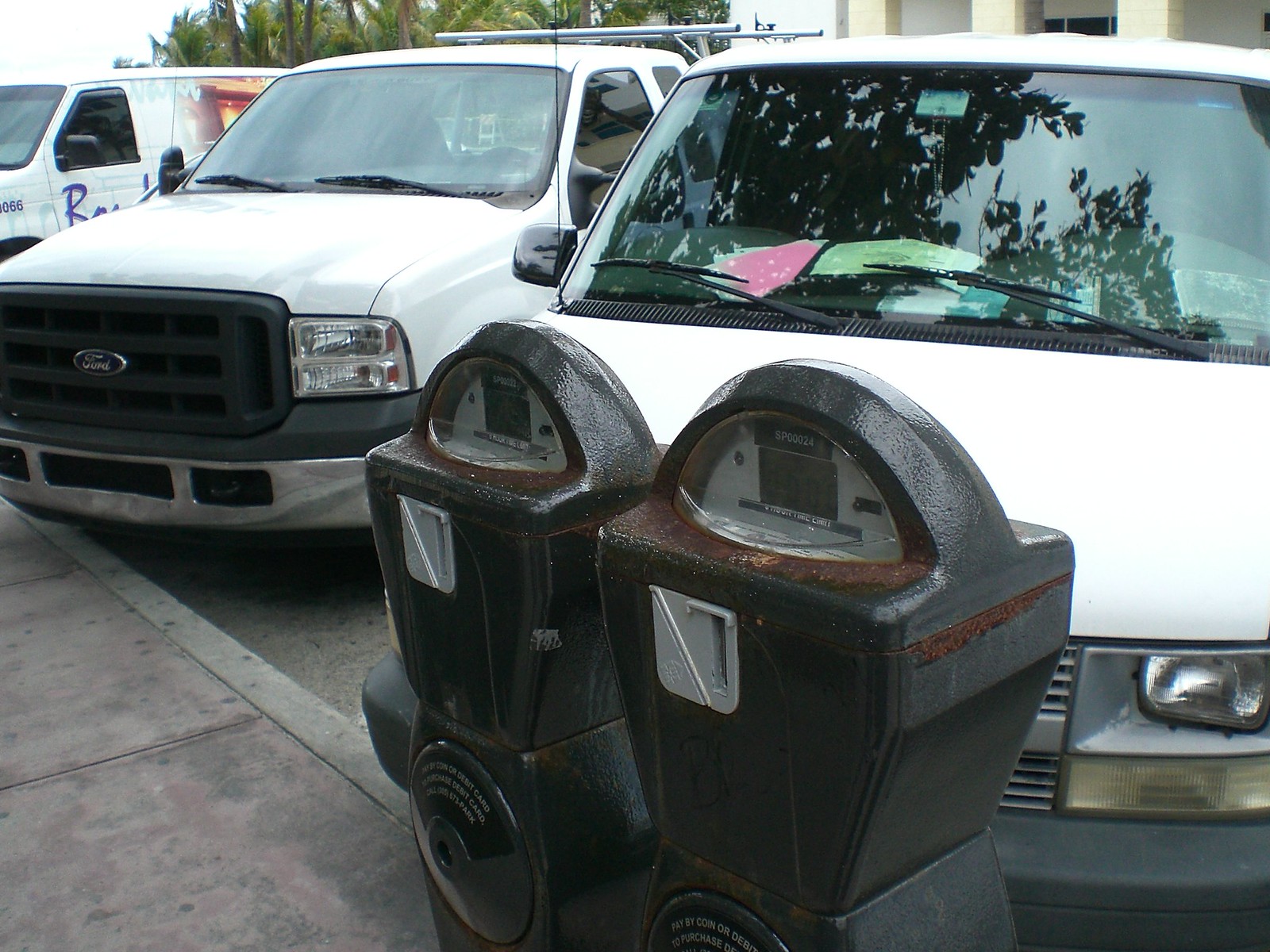This color photograph captures an outdoor parking lot scene with a pair of old-fashioned, gray parking meters prominently in the foreground. The parking meters are side by side, showing signs of rust around the meters and above the coin slot. Each meter features a digital display under a glass cover. In the background, three white vehicles are angle-parked: 

1. **Closest to the foreground**: A white van, with the windshield reflecting nearby trees. Papers in pink, green, and blue are visible on its dashboard.
2. **Middle vehicle**: A white Ford pickup truck, identifiable by its black grille and a metal rack mounted on the back.
3. **Furthest vehicle**: Another white van with partial writing starting with "R" on the driver’s side door.

All vehicles have clear windshields, black windshield wipers, and black antennas. Beyond the vehicles, one can observe trees and part of a white building, along with a patch of sky that is bright and mostly white. The scene is well-lit, with the glare of sunlight evident on the closest van. The pavement in front of the parked vehicles is a plain gray sidewalk.